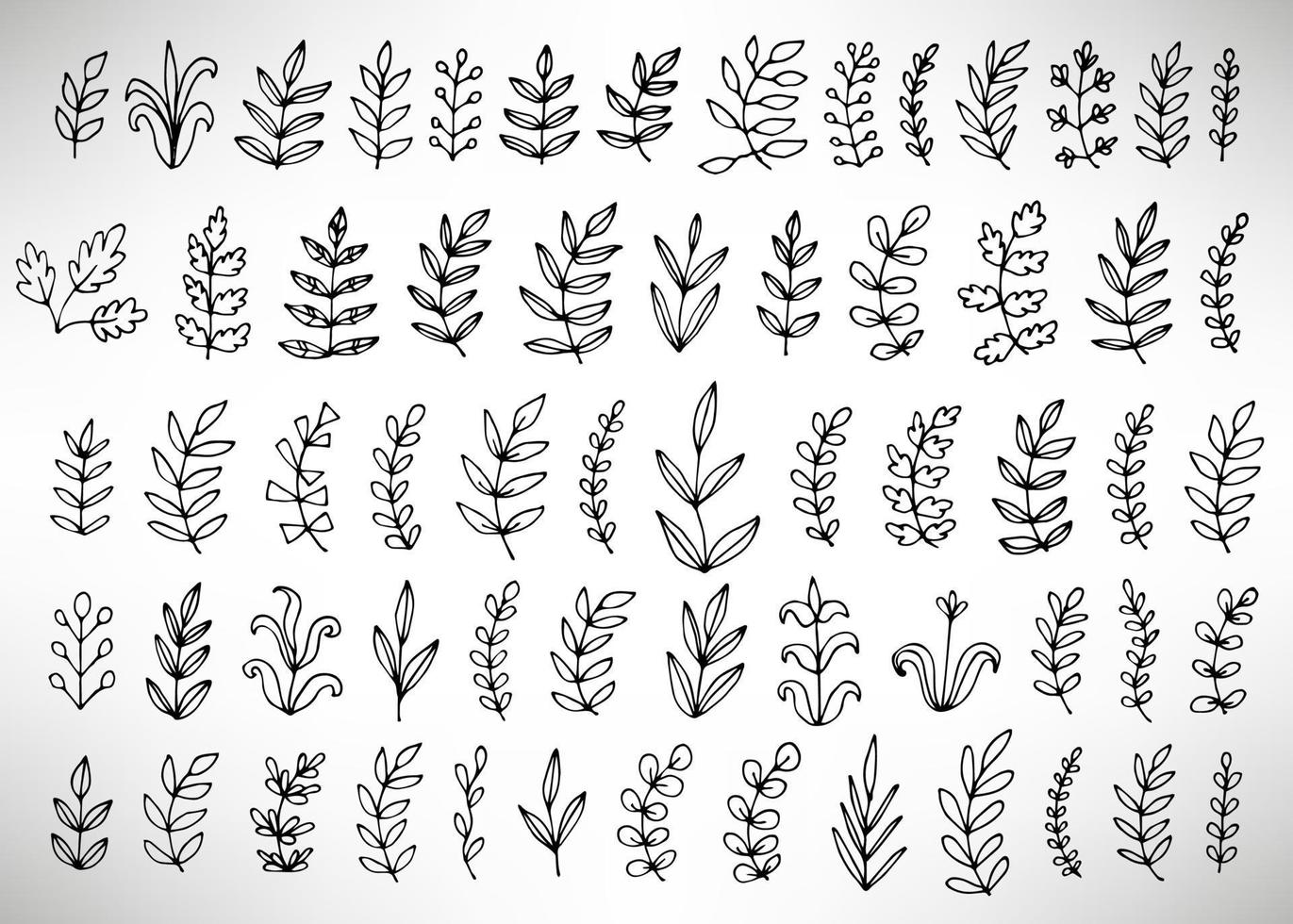This hand-drawn design in black ink on a white sheet features an intricate array of small plant illustrations meticulously arranged in a landscape orientation. There are 5 horizontal rows, each containing 14 unique drawings of delicate plant stems, totaling 70 individual plant pieces. Each stem displays varied and meticulously detailed leaf formations—some with a dozen leaves, others with just five or fewer. The leaves themselves vary significantly in shape, ranging from almond and oval shapes to tiny sticks with ball-like structures or curvy leaf designs. Despite some similarities, every plant illustration remains distinct, showcasing a rich diversity of styles and forms. This collection, reminiscent of a botanical study, provides a fascinating visual exploration of plant morphology.